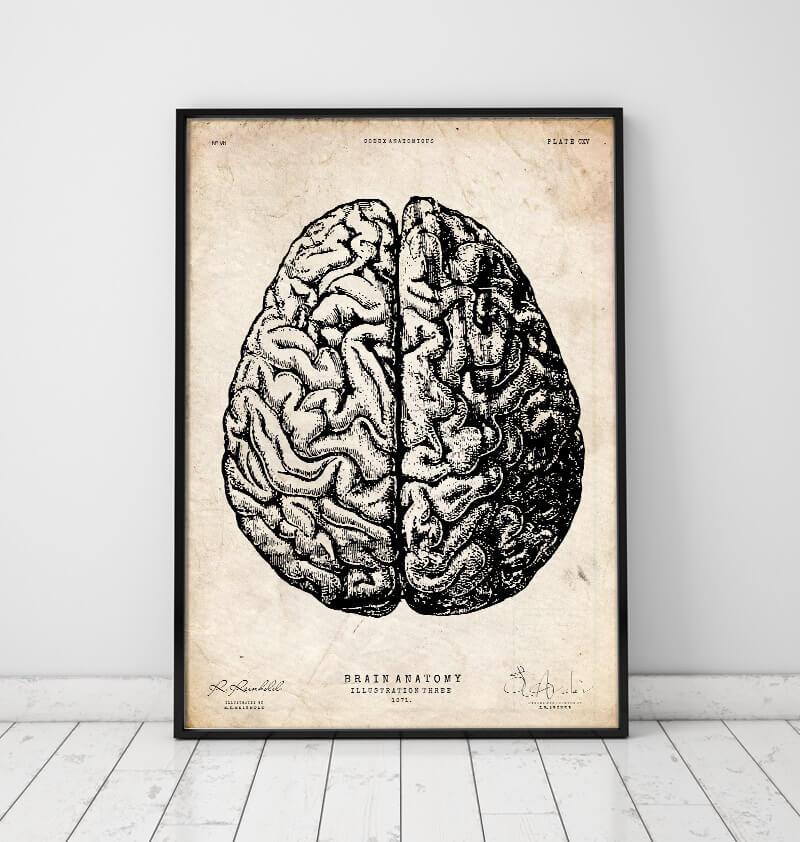This is a detailed black-and-white painting of a brain, prominently displayed in a vertically aligned rectangular picture frame with a thin black border. The brain is depicted with its center slightly cracked open. The background of the painting has the appearance of a faded, old piece of paper, giving it a beige or tan color, akin to aged parchment. At the bottom of the painting, the text reads "Brain Anatomy, Illustration 3TL," although some characters are unclear. There are two signatures: one on the lower left, which is faded and difficult to read, and another on the lower right. The painting is leaning against a white wall with an older-looking, marked baseboard. It is placed on a gray floor that appears to be composed of vertical strips of white wooden tiles, which may have a marbled or scratched appearance.